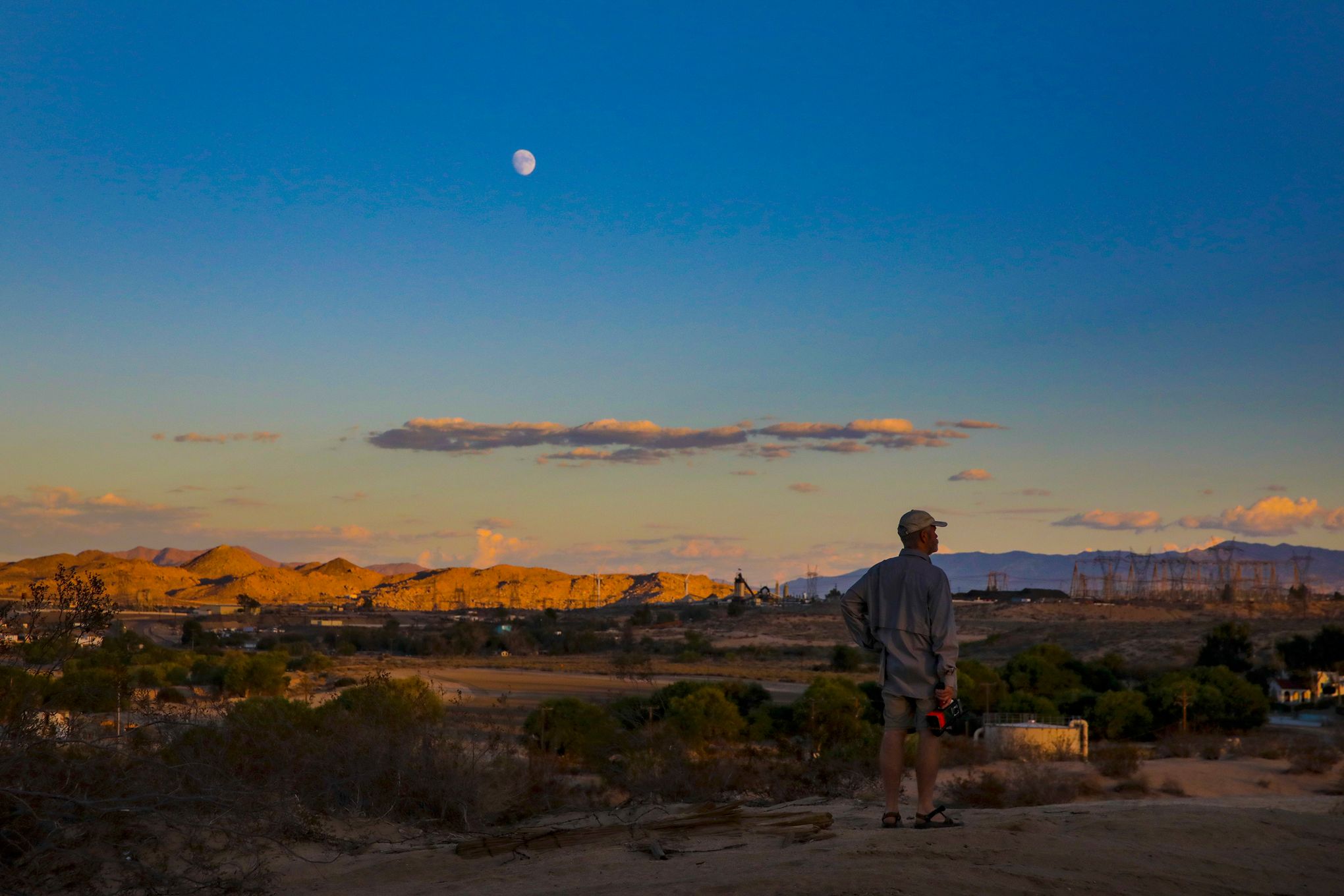In this captivating dusk photograph, a man stands in the foreground of a desert landscape, dressed in shorts, black sandals, a long-sleeved blue jacket or shirt, and a white baseball cap. He holds a flashlight or radar gun in his right hand and has his left hand propped on his hip as he gazes towards the right. The ground beneath him is dry dirt or sand, scattered with small desert plants and scrubby bushes. The scene features a neighborhood of houses in the middle distance, leading up to a stunning backdrop of sunlit desert mountains glowing golden with hints of blue. The sky above is a deepening blue adorned with wispy white clouds, the moon peeking through, and the last rays of the setting sun contributing a touch of warmth. The entire foreground is shadowed, contrasting with the illuminated mountains in the distance, encapsulating the serenity of the transition from day to night.